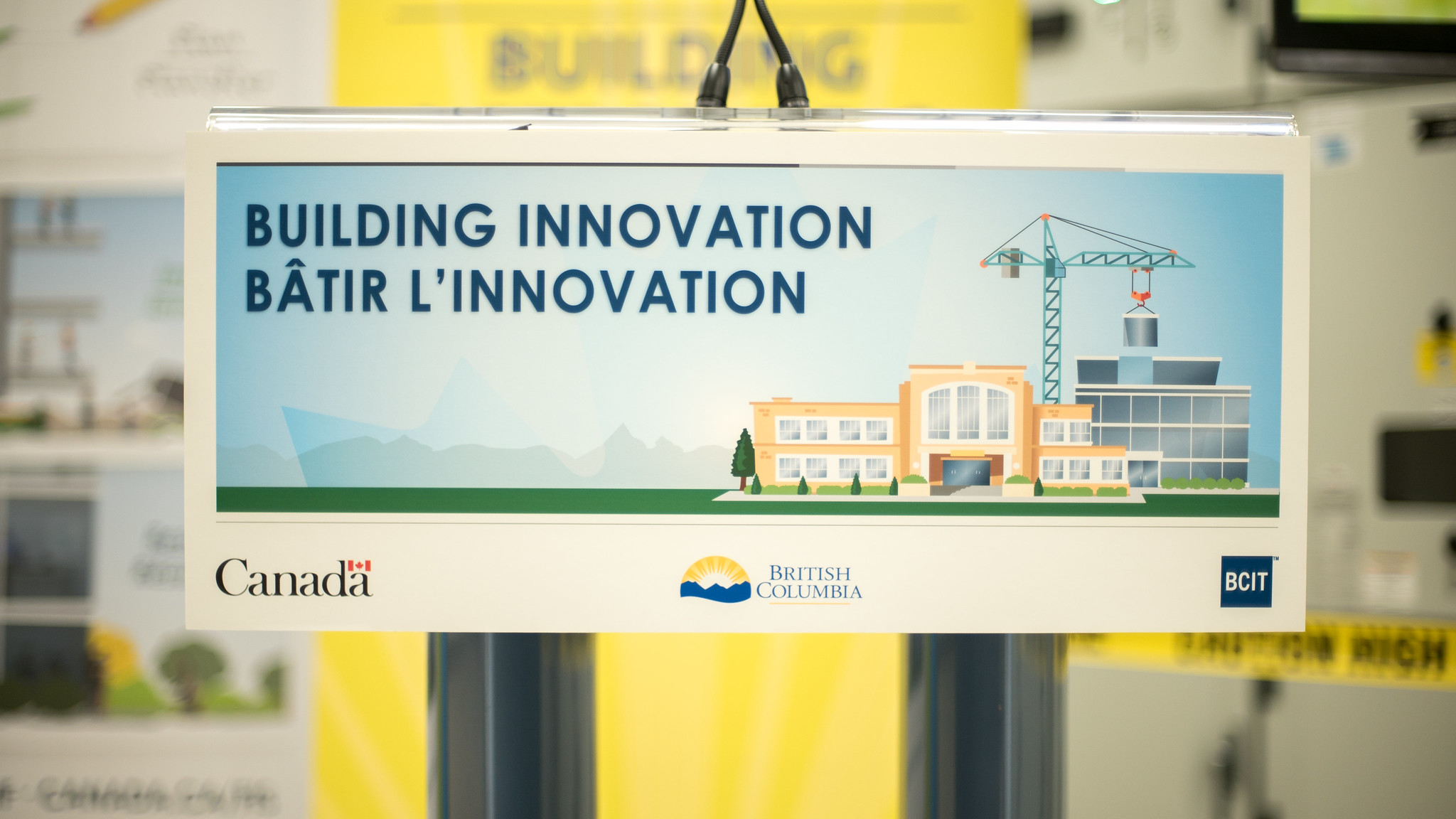The image features a small, white sign suspended by two closely spaced black wires. The sign is set against a backdrop that suggests an outdoor event, possibly related to construction or a conference, indicated by blurred banners and a strip of yellow construction tape. The main focus of the sign includes:

- **Top Left**: The word "Canada" with a small Canadian flag above the final 'A'.
- **Center Bottom**: The text "British Columbia" beneath a blue silhouette of a mountain and a yellow half-circle representing the sun.
- **Bottom Right**: A dark blue box containing the acronym "BCIT".
- **Central Image**: A light brown, two-story building with windows. Beside it, an animated construction crane lowers a silver cylinder onto another building with a glass front.
- **Text**: The phrase "Building Innovation" appears prominently, with its French translation, "Bâtir et l'Innovation", beneath it.
- **Background**: The sky transitions from blue on the right to a lighter yellowish-white hue on the left. 

The scene depicted suggests ongoing construction, with an emphasis on innovation and development in British Columbia, Canada.